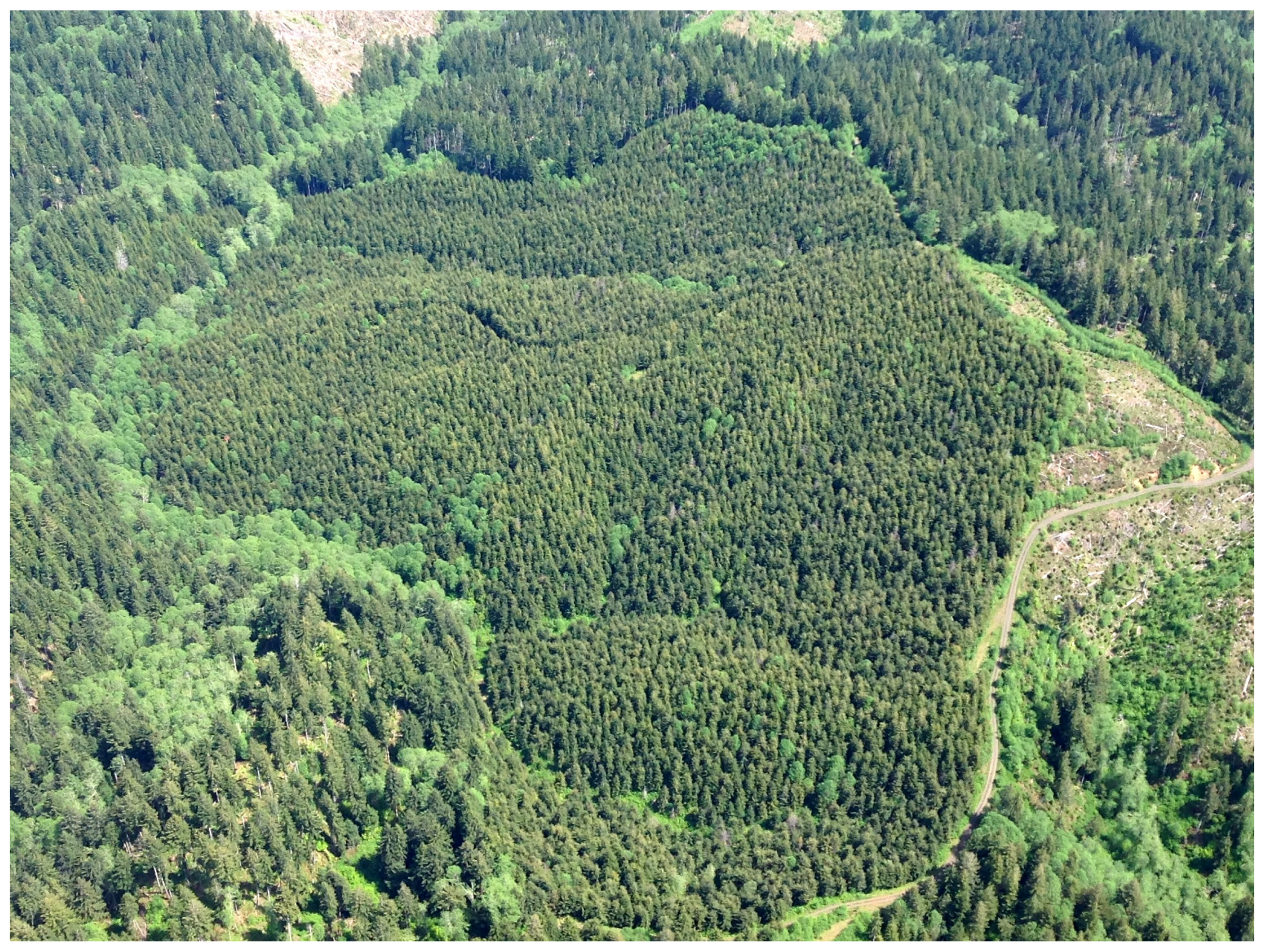The image captures a stunning aerial view of a dense, expansive forest from a very high altitude, possibly taken from a helicopter, plane, or drone. The entire scene is bathed in natural daylight, showcasing vibrant colors and clear details, indicative of a bright, sunny day. 

The forest is composed of a mixture of trees, with varying shades of green: some are a lighter hue, while others are a deep, dark emerald green. The trees are so densely packed that the ground is completely obscured in most areas. In the bottom right corner of the image, a winding roadway is visible, likely a gravel road, though it appears devoid of any vehicles. 

Additionally, there are patches of stone visible in the top sections of the image, suggesting a varied terrain. The lush green grass further complements the thick foliage, emphasizing the richness of this natural setting. The image is devoid of any human presence, words, or numbers, purely focusing on the beauty and density of the forested area, possibly located in the Northwestern United States.